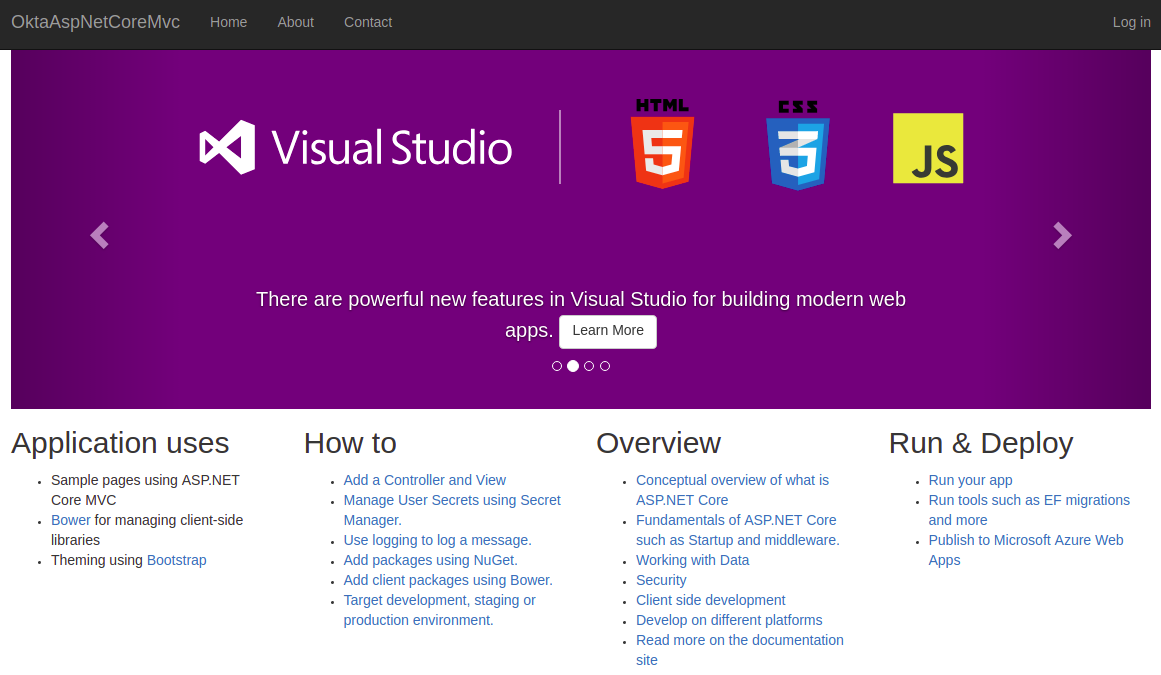The image is a visually structured webpage design mockup that is approximately 50% wider than it is tall. At the top, there is a sleek black header bar that spans the width of the image, occupying about 10% of the image's height. In this header, positioned on the left in gray text, is a lengthy site name reading “Okta AspNetCoreMVC” without spaces. To the right of this text are three navigation menus labeled "Home," "About," and "Contact." At the far-right corner of the header, there's a "Log In" option, also in gray text.

Beneath the header, the background transitions to a smooth plum purple gradient, slightly lighter towards the center and darker at the edges. About one-third down the image, there is a prominent Visual Studio icon accompanied by the text "Visual Studio," both in white. To the right of the Visual Studio text, separated by a vertical white line, are three notable icons lined up horizontally. 

The first icon is the HTML5 logo, depicted as a stylized shield with an orange background, containing a white "5" symbol. Next is the CSS3 logo, also in the shape of a shield but with a blue background and a white "3" symbol. The final icon in this series is for JavaScript, featuring a vibrant yellow background with the "JS" letters in black.